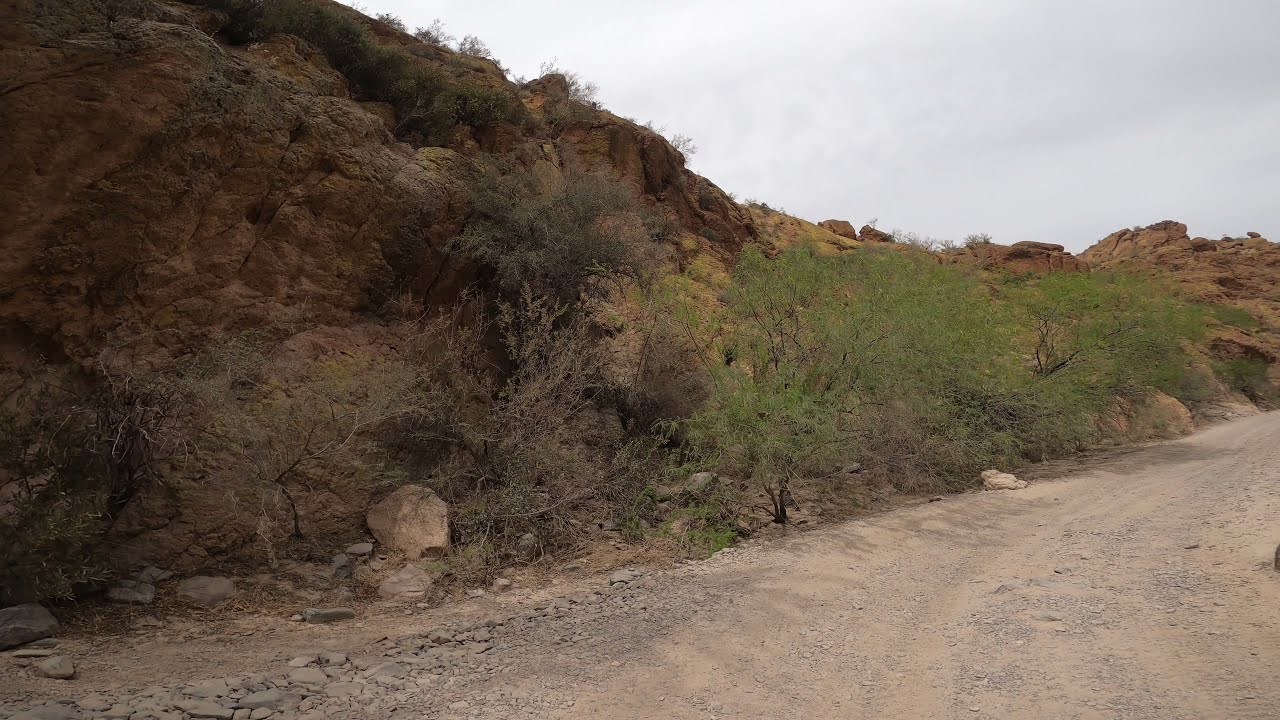This is an outdoor photograph depicting a desolate and rugged desert landscape. In the foreground, a beige, unmetalled dirt road curves towards the right, with grey pebbles scattered about its surface. Adjacent to the road on the left is a small cliffside, composed mainly of tan and brown rocks interspersed with stunted shrubs and bushes. These sparse plants vary in color, with some showing patches of green amidst predominantly grey and brown hues, indicating dryness. The overall surroundings appear barren and dry, enhancing the stark, arid atmosphere of the scene. Overhead, the sky is overcast, blanketing the landscape in a somber grey, suggesting a midday setting without direct sunlight. The distant rocky expanse maintains the same rugged and dry characteristics, solidifying the image as one of stark desert isolation.